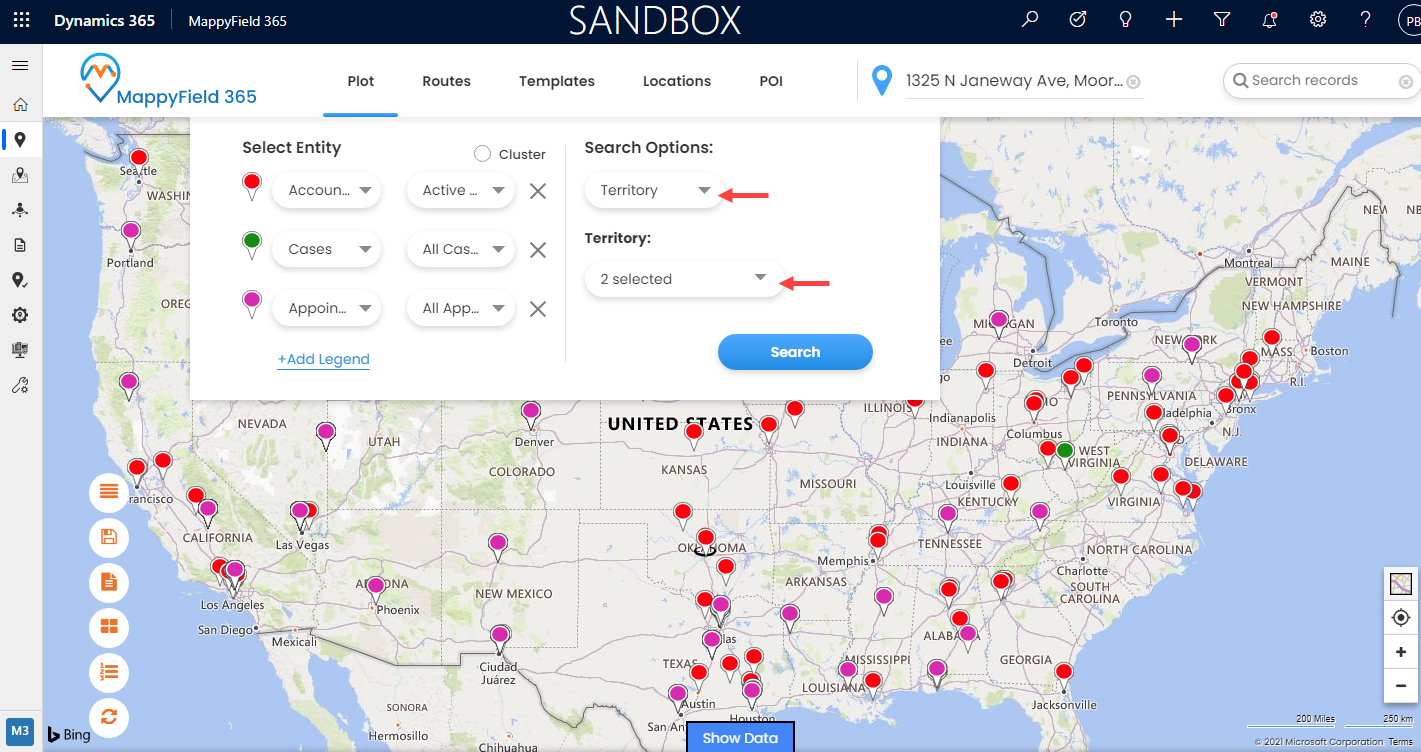The web page features a background map of the United States, dotted with numerous red pinpoints. Dominating the top of the image is a black rectangular box stretching from left to right. Centrally positioned within this black box is the word "Sandbox" rendered in white text, possibly indicating the name of the page. Slightly below, there's a logo composed of a blue pinpoint with an orange "M" inside it, adjacent to which is the text "Mappy Field 365" in blue, suggesting another potential name for the web page.

In the top-left center of the image, there's a prominent white box filled with various icons and labels. This box is titled "Select Entity." Below this title, there are three colored pinpoints: a red one labeled "Account," a green one labeled "Cases," and a purple one labeled "Appointments." Each pinpoint is selectable. To the right of this white box, the title "Search Options" is displayed. Under this heading, "Territory" appears as an option at the top, followed by another "Territory" label below it. The box beneath these labels includes an adjustable selection labeled "To Selected." Finally, at the bottom-right of this section, a blue oval button with the text "Search" in white stands out, indicating its function.